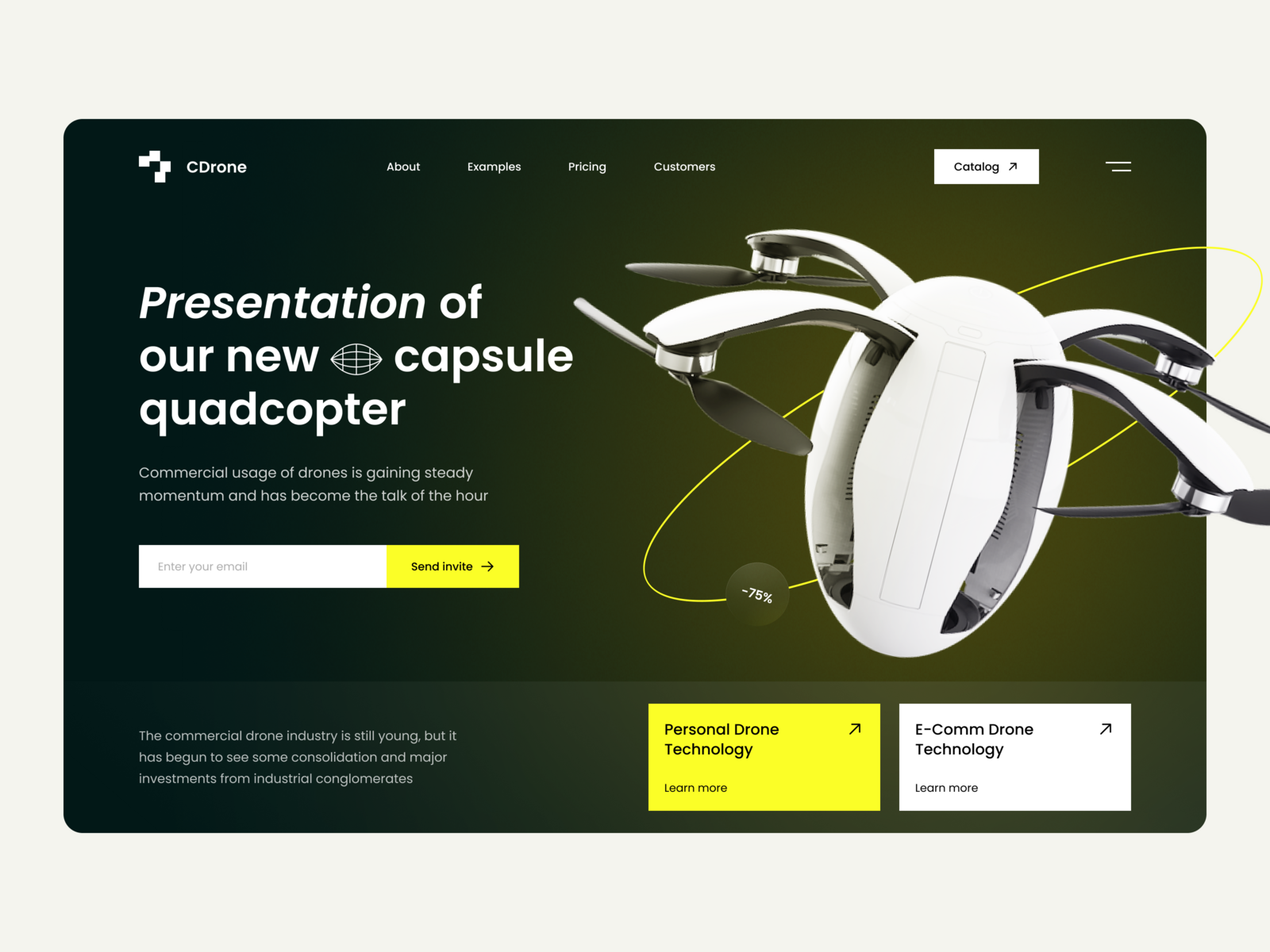This is a screenshot of a product website featuring a sleek and modern dark green design. At the top-left corner, the company's logo, "CD-Drone," is prominently displayed. To the right of the logo, a top navigation menu features four white text links labeled "About," "Examples," "Pricing," and "Customers." Further to the right, a rectangular button labeled "Catalog" with an upward arrow icon is positioned, also in white. Below this navigation bar, large white text on the left side of the screen announces, "Presentation of our new capsule quadrocopter." Just beneath this headline, smaller text explains, "Commercial usage of drones is gaining steady momentum and has become the talk of the hour." Dominating the lower portion of the screen is a large photo of the quadrocopter, which boasts a unique, egg-shaped body and four rotors, highlighting its innovative design.